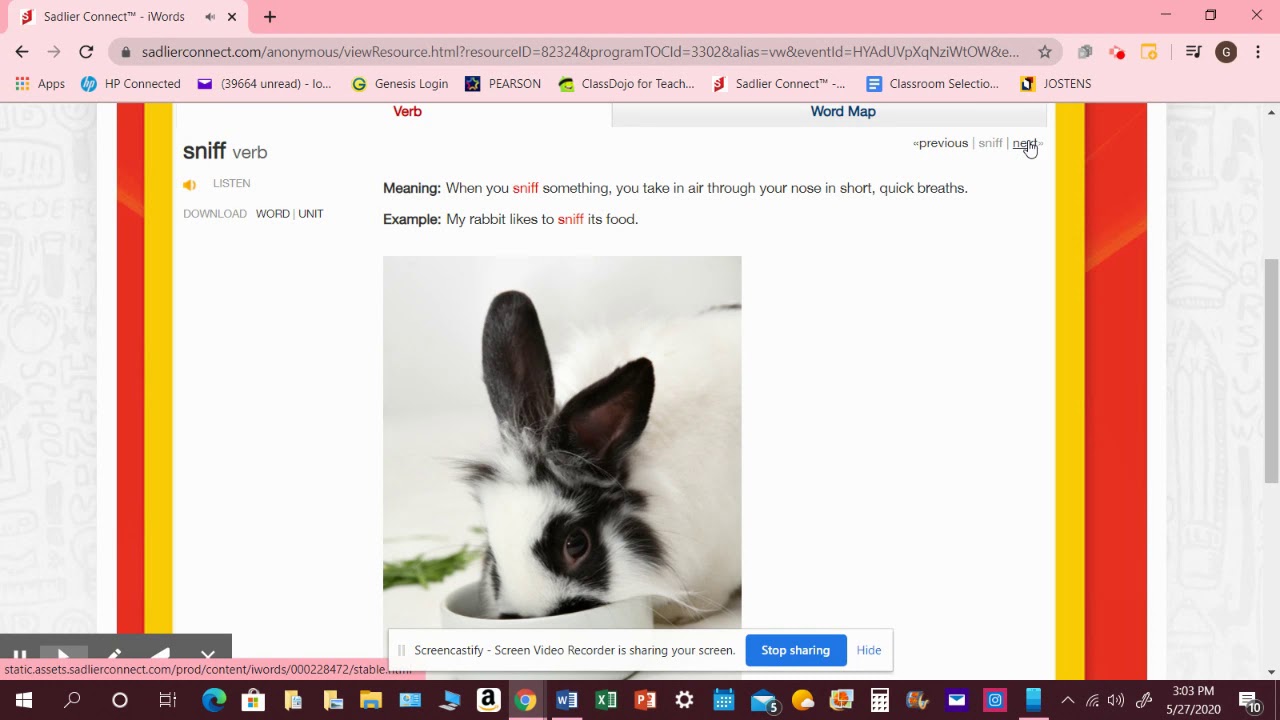The image depicts a screenshot of a detailed and somewhat cluttered educational website accessed on a Windows computer. Noteworthy features are as follows:

- **Operating System**: The image was captured on a Windows computer, evident from the distinct Windows taskbar at the bottom, which includes icons like the Chrome browser, Amazon One, various Microsoft Office applications, and a Calculator among others. The time displayed on the taskbar indicates it is 3:09 PM on May 27, 2020.

- **Browser Details**: The current open tab on the browser displays the website "SaddlerConnect.com", visible in the address bar accompanied by a long string of alphanumeric characters. The browser's user interface includes a pink-colored toolbar atop.

- **Website Content**: Central to the webpage is an educational section featuring the word "sniff" as a verb. The definition provided explains that 'to sniff' involves taking air through the nose in short, quick breaths. An example sentence, "My rabbit likes to sniff its food," is provided in red text. Adjacent to the text is an image of a predominantly white rabbit with black ears and markings around its eyes. The rabbit is shown next to a white food bowl on a white background, with some green leaves to the left of it.

- **Layout and Border**: On either side of the main content are two grey bars which have a pencil watermark effect, appearing somewhat old-fashioned or dated. An orange bar, thicker on the left than the right, and a yellow bar also frame the content.

- **Top Navigation**: The top navigation bar lists other areas such as HP Connect, unread emails, Genesis login, Pearson, and Class Dojo for Teach.

- **Screen Interface Elements**: The bottom right of the screen indicates the presence of Screencastify, a screen video recording application informing the user that screen sharing is active with the option to stop sharing or hide the notification via a blue button.

This highly detailed representation suggests a focus on educational content, likely aimed at young students, within a user interface that combines various navigational and illustrative elements.